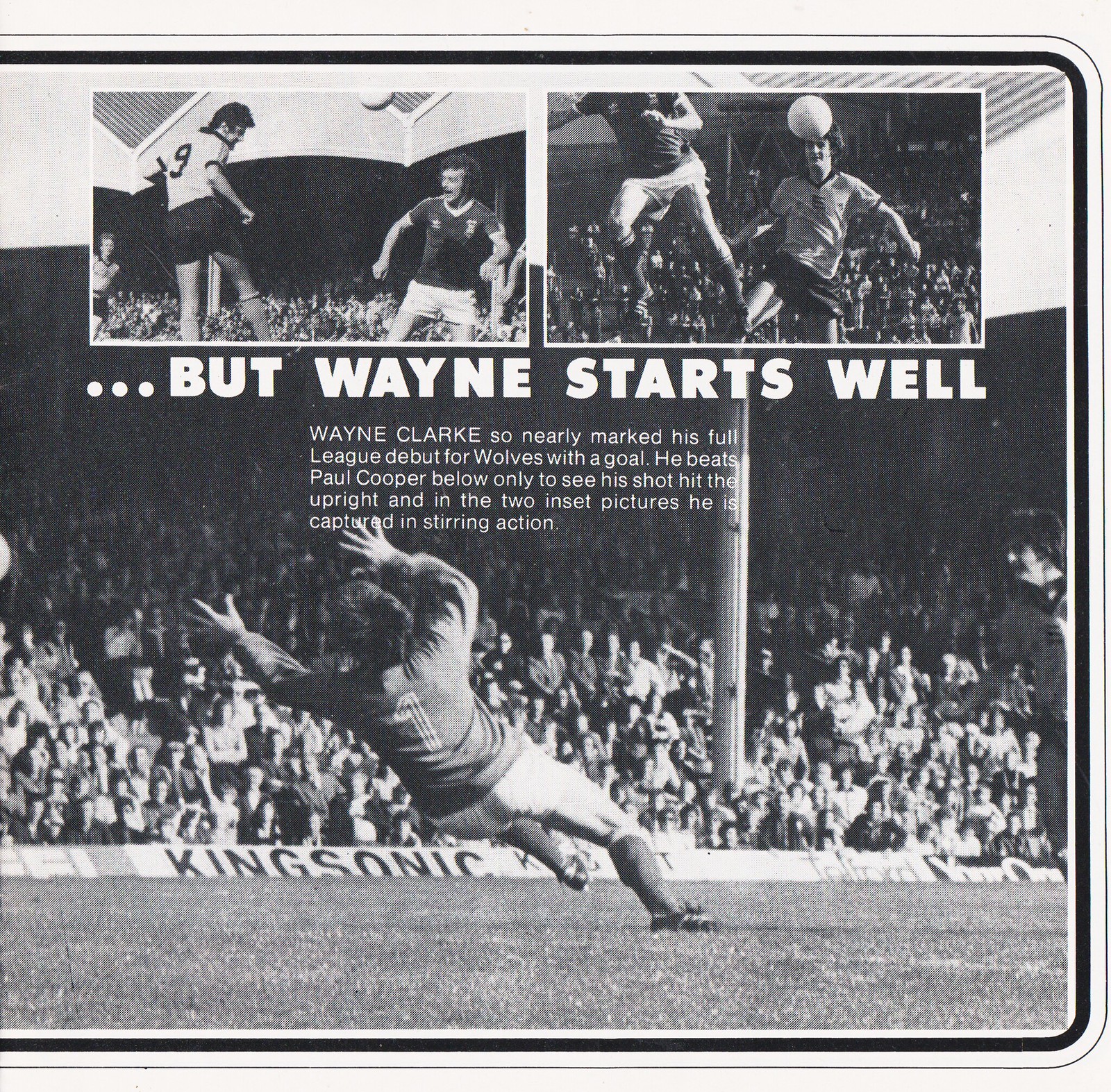The image depicts a black-and-white page from a sports magazine or newspaper, featuring a detailed layout centered around three dynamic soccer snapshots. The central image dominates the lower two-thirds of the page, capturing a dramatic scene with a soccer player diving to make a save or potentially score, amidst an attentive crowd in the bleachers. Above this main action shot, the top third of the image hosts two inset photos: one showing a player heading the ball and the other depicting a goalkeeper poised to block an incoming goal. The text overlays provide context, highlighting Wayne Clark's near-marking debut for the Wolves, describing how he narrowly missed scoring when his shot hit the upright. All elements are rendered in shades of black, white, and gray, emphasizing the intensity and historical value of the moment captured.